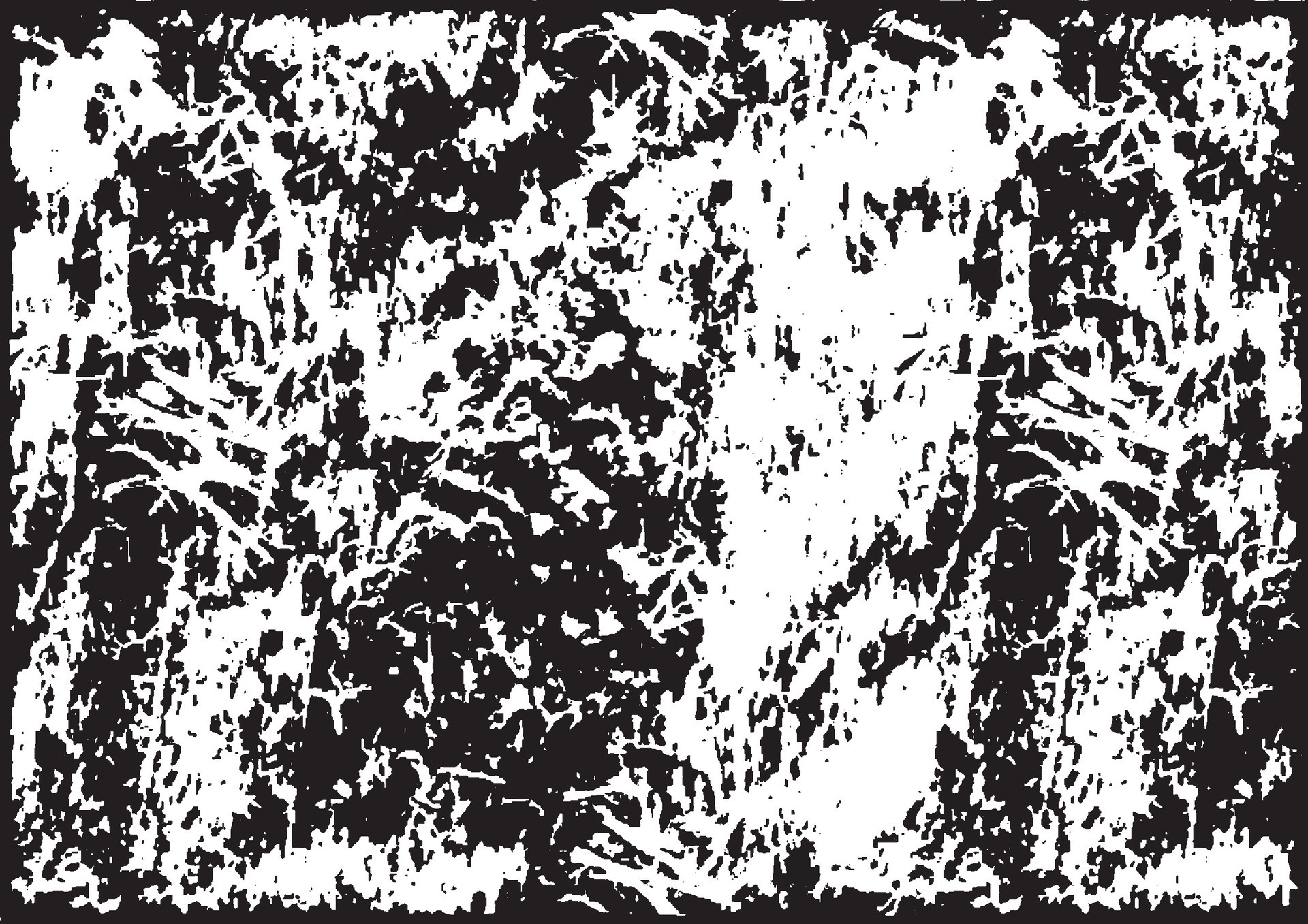This image is a highly abstract digital artwork resembling a pixelated woodcut, created entirely in black and white. The composition features an intricate arrangement of black pixelated dots, scribbles, and streaks against a contrasting white background. The artwork appears to be evenly balanced between black and white areas, though there may be a slight emphasis on the black portions, especially around the edges where the black is more pronounced.

At the center, the white areas form chaotic patterns, with some parts resembling Z-shaped scribbles that suggest repetition on both the left and right sides of the image. These repeating patterns lend the piece a sense of symmetry, despite its overall chaotic appearance. Among the abstract forms, some shapes hint at tree-like figures, potentially appearing as spooky or surreal objects on both sides of the image.

The image lacks any text or explicit narrative, leaving its interpretation open to the viewer. As an engaging piece of art, it successfully captures the essence of abstract expressionism, requiring the audience to delve into its intricate patterns and forms.